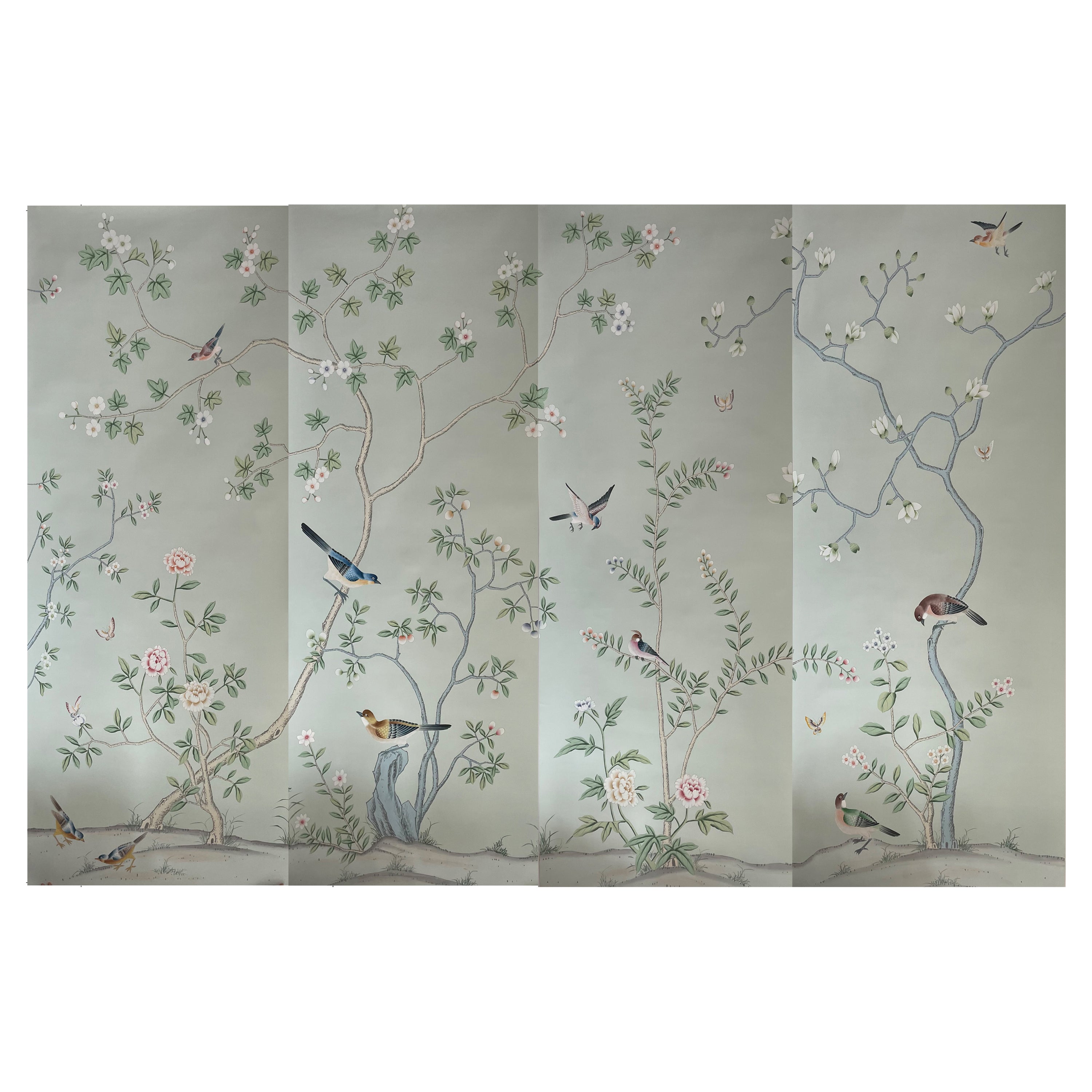This photograph depicts a continuous four-panel artwork that functions as a privacy screen, each vertical panel seamlessly connected with visible folds. The background is a serene, pale gray, providing the perfect backdrop for a delicate nature scene inspired by Japanese aesthetics. Slender branches and tree trunks adorned with white and pink blossoms and green leaves extend upwards, creating a lush botanical tapestry. Scattered among the branches are a variety of vividly detailed birds. Notable avian figures include blue and brown birds, one with a white underbody, and two birds caught in flight—one in the top right and another descending in the center. In the bottom left corner, two birds peck at the ground, possibly searching for seeds. The overall composition, with its taupe hues and floral accents, evokes a sense of tranquility and quiet beauty.